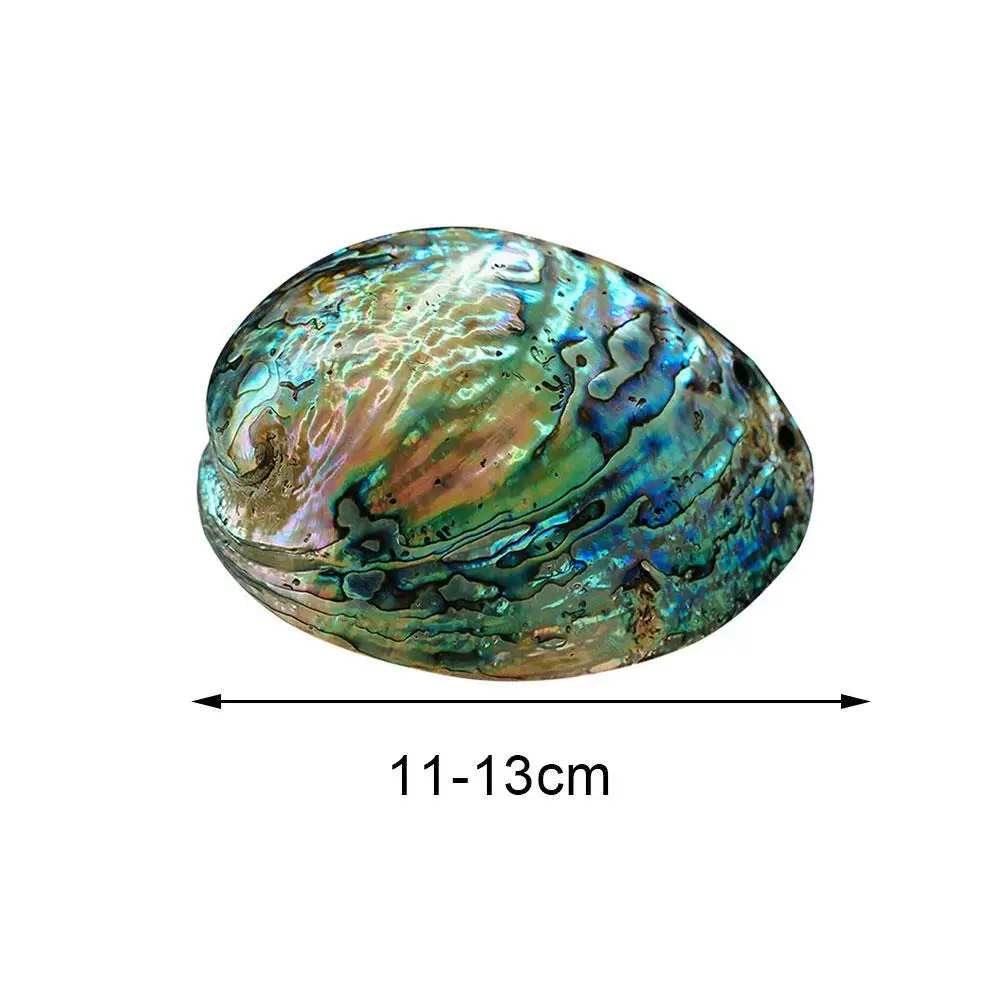The image features an abalone shell as the focal point, beautifully displayed against a plain white background. The shell is domed and somewhat slim, showcasing a multicolored, rainbow-like, and metallic appearance with a predominantly smooth but subtly rippled surface. Hues of blue, green, pink, and orange interlace, giving it a pearly, iridescent sheen. Beneath the shell, a thin black arrow extends left and right, matching the shell's length, approximately 11 to 13 centimeters, as indicated by the scale below the arrow. The shell's detailed depiction makes it difficult to discern whether it is an actual shell or a digitally generated image.